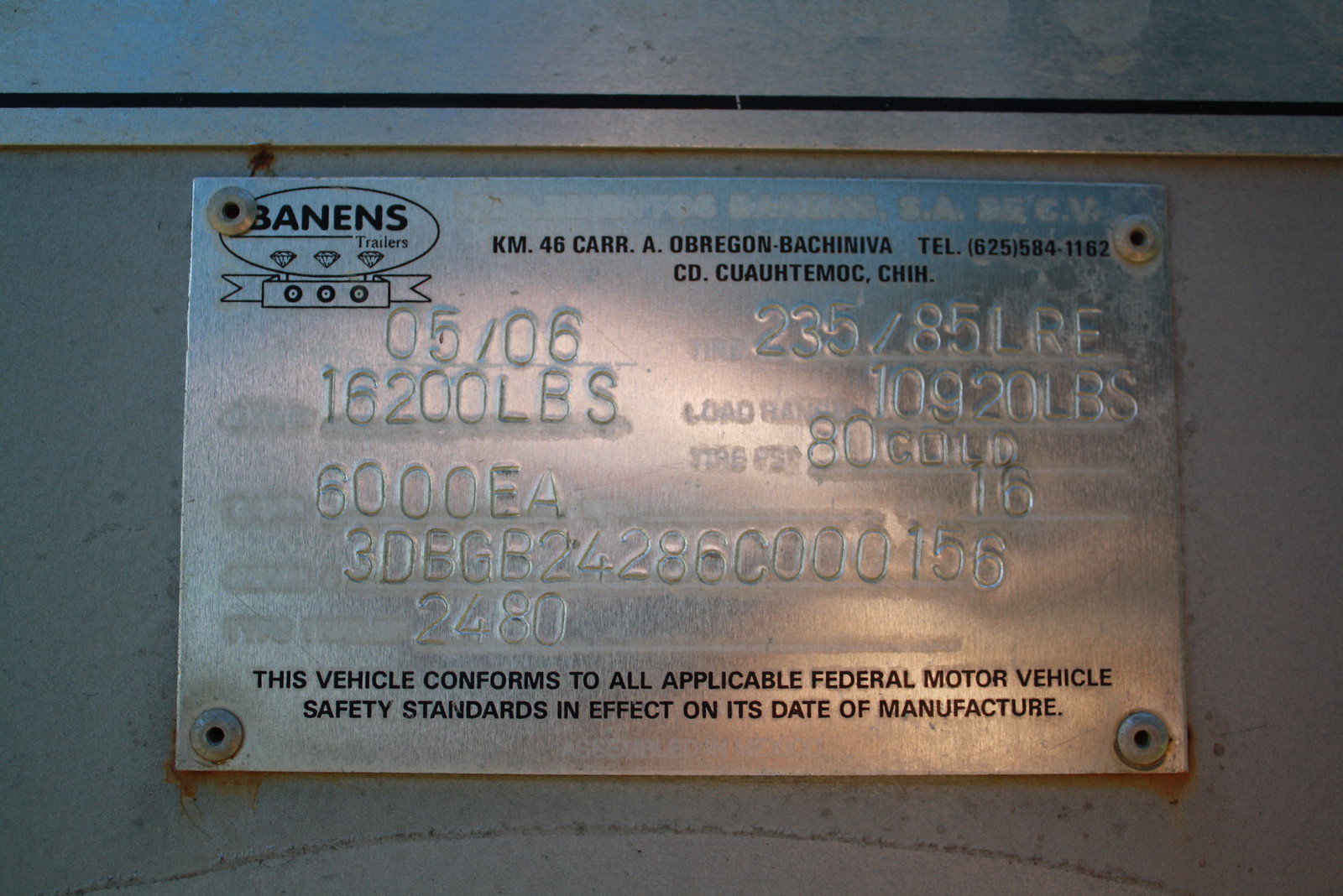The image depicts a silver metal plate affixed to a gray wall with screws at each of its four corners. The upper left corner of the plate features the logo "Ben & Strader's" (alternatively referred to as "Baninj Trailer" or "Bannens Trailers"), though the correct spelling appears to be "Ben & Strader's." Below the logo, various numbers are prominently embossed, including the sequence "05/06," "16,200 pounds," and "6,000 EA." These numbers occupy the central portion of the plate. At the bottom, there's a critical certification notice stating, "This vehicle conforms to all applicable Federal Motor Vehicle Safety Standards in effect on its date of manufacture." Additional contact information is etched into the top right corner, displaying the telephone number "625.584.1162." All inscriptions and numbers appear in an uncolored, embossed format.